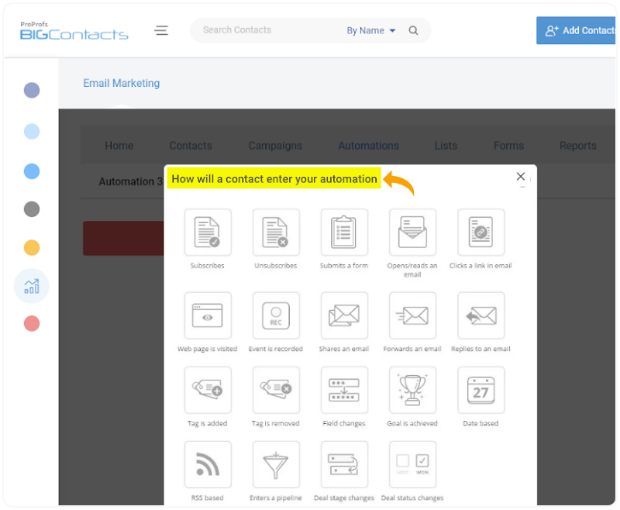The image is a detailed screenshot of the "Big Contacts" interface, showcasing a variety of automation triggers for managing contacts. The background is grayed out, while a prominent white pop-up window is in focus. At the top of the interface, there are search options available for finding contacts by name, adding contacts, and managing email marketing. 

The pop-up window is titled "How will a contact enter your automation?" and this section is highlighted in yellow, drawing attention through an orange arrow pointing directly at it. Beneath this highlighted area, an array of icons represents different automation triggers:

- **Subscribes**: Represented by a paper icon.
- **Unsubscribes**: Identified with a similar paper icon.
- **Submits a form**: Indicated by a clipboard icon.
- **Opens/Reads an email**: Marked by an envelope icon.
- **Clicks a link in an email**: Displayed as a page icon.
- **Web page is visited**: Shown with a browser icon.
- **Event is recorded**: Signified by a record button icon.
- **Shares an email**: Depicted with a double envelope icon.
- **Forwards an email**: Illustrated by an envelope icon with speed lines emanating from the left side.
- **Replies to an email**: Denoted by an envelope icon with an arrow pointing to the left.
- **Tag is added**: Shown as a price tag icon.
- **Tag is removed**: Represented by a price tag icon with an 'X' on it.
- **Field changes**: Visualized with an icon of two field bars.
- **Deal was advertised**: Denoted by an icon of a glittering trophy.
- **Date based**: Represented by a calendar icon marked with the number "27".
- **RSS based**: Indicated by an RSS feed icon.
- **Enters a pipeline**: Depicted with a funnel icon.
- **Deal stage changes**: Illustrated by an icon of two search bars.
- **Deal status changes**: Shown as an icon with two check boxes, one of which is checked.

This comprehensive array of icons and their corresponding actions illustrate the flexibility and depth of the automation capabilities within the "Big Contacts" platform.